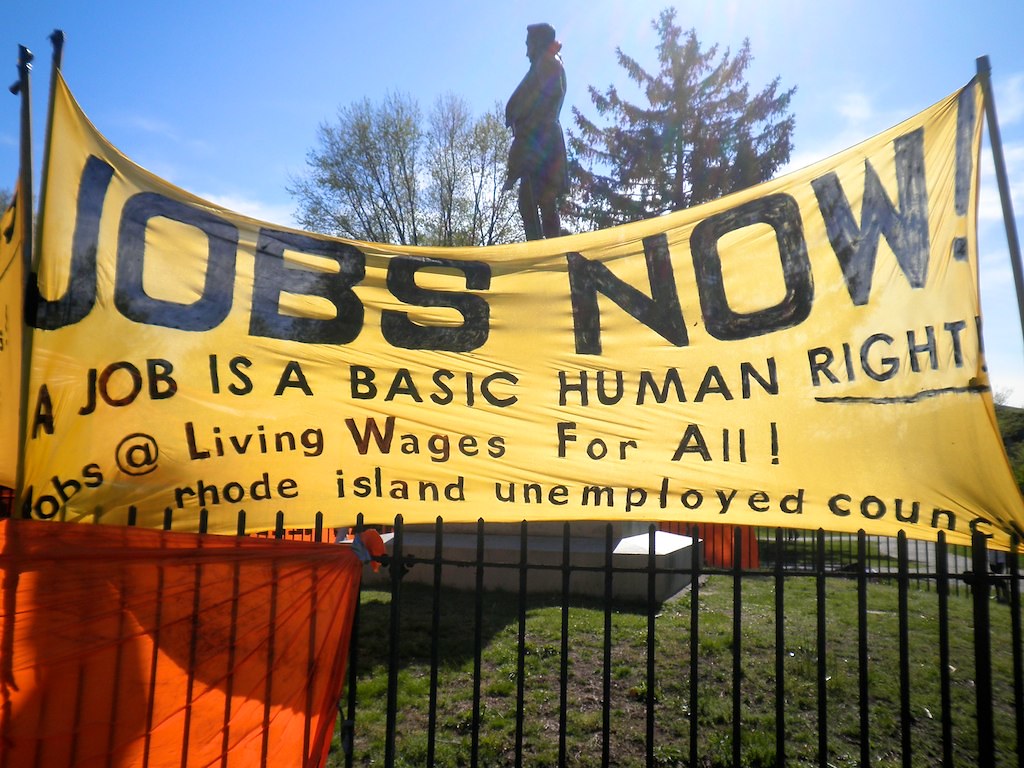In the foreground of this vibrant color photograph, a wrought iron fence occupies the lower third, adorned with a red tarp tied to the left side extending outward. Above the fence, a prominent yellow banner stretches between two black poles, though it sags slightly. Bold black text on the banner declares, "JOBS NOW!" with an exclamation mark. Below, it reads, "A job is a basic human right," with "right" underlined, followed by, "Jobs at living wages for all," and finally, "Rhode Island Unemployed Council." Beyond the fence lies a grassy area leading to a granite platform supporting a statue of a historical U.S. figure, likely from the 17th century. The scene is framed by two trees—one a pine and the other with small leaves gently falling. Above, the sky is a brilliant blue, dotted with wisps of white clouds.